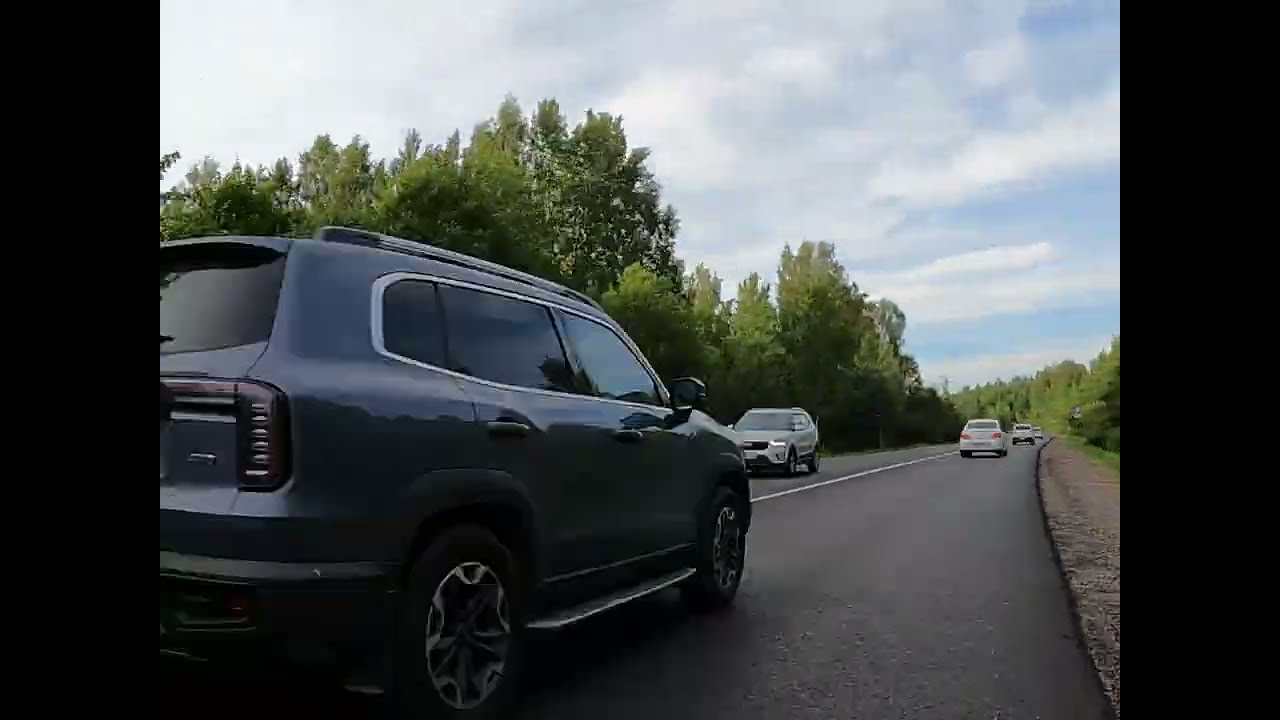The image captures a clear day on a rural, forested two-way road made of black asphalt. There are trees and greenery lining both sides of the road and a small shoulder on the right side. At the top of the image, the sky is a vibrant blue scattered with white clouds. Closest to the viewer, on the left side, is a dark SUV (likely black or very dark blue) with interesting wheels and a hatchback, appearing to travel at a regular speed. On the opposite side of the road, a silver SUV is approaching. Further ahead, two white cars are visible in the same lane as the dark SUV, and another white car can be seen further down the road. There are no visible obstructions or accidents, and the scene is relatively uncrowded, yet one must still heed the speed limit. The cars, the trees, the sky, and the road are predominantly colored in shades of white, blue, green, gray, silver, brown, and red.